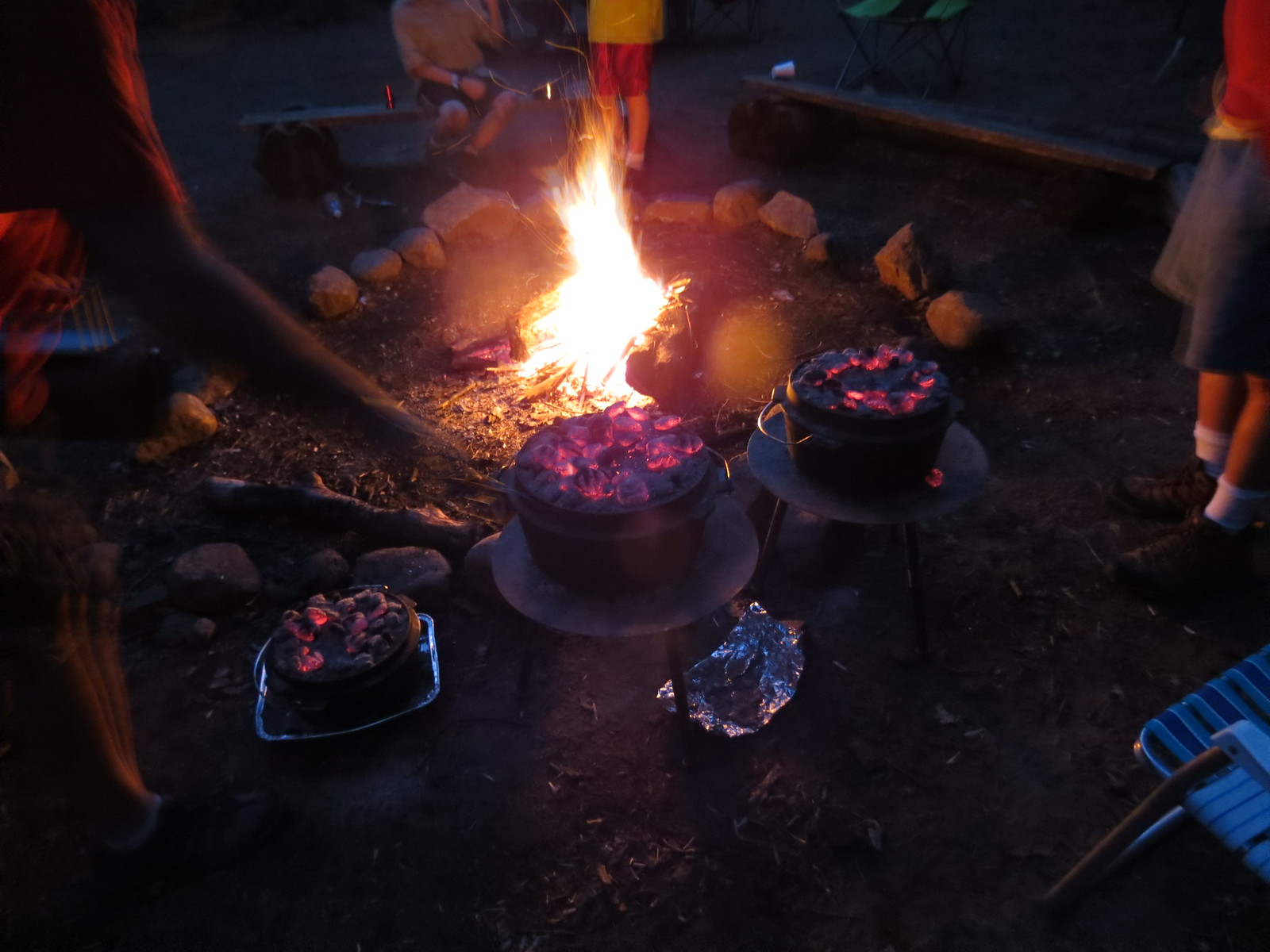This image depicts an outdoor campfire surrounded by a variety of elements and activities. At its center, the fire blazes within a pit encircled by small stones. Surrounding the fire pit are several figures and objects contributing to the evening's scene.

On one side of the campfire stands a person wearing gray shorts, white socks, and black shoes. Adjacent to them, another individual is visible with blue shorts, possibly red top, tan legs, and white socks paired with black shoes, creating a silhouette against the flickering flames. Additionally, there's another figure in dark shorts and a tan long-sleeved shirt with rolled-up sleeves, their arm bent as if in mid-action, perhaps eating or drinking.

To the right of the fire, two tables hold pots filled with glowing red coals. One of these tables is short and wooden, while the other appears to be a simple metal frame. A piece of discarded aluminum foil lies beneath one of these tables, adding to the casual, lived-in atmosphere of the scene. Nearby, a foil pan also contains hot coals, contributing further to the communal warmth.

In the background, a bench rests with what looks like a can of Dr. Pepper or Coke placed upon it. The edge of a blue and dark blue lawn chair with a rusty metal base can be seen in the bottom corners of the image, hinting at more seating scattered about. Sticks and wood chips are scattered around, and some parts of the scene appear slightly blurry, emphasizing the focus on the crackling campfire and the people enjoying it.

Overall, this image captures a social gathering around a campfire, with details like glowing coals, casual seating, and the presence of friends or family making it a warm, inviting scene.